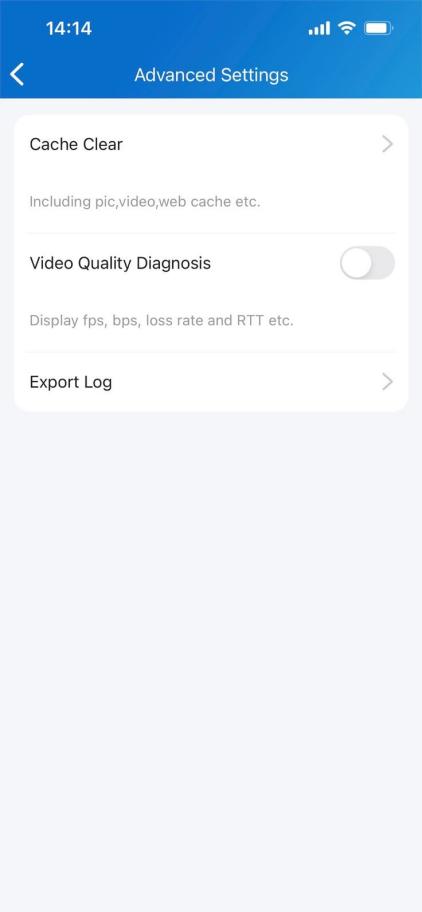The image is a screenshot from a mobile device's advanced settings menu. At the top, a blue bar stretches horizontally across the screen. On the left side of the blue bar, white text displays the time "14:14," indicating 14 minutes past 2 o'clock. On the right side of the bar, icons show the device's connectivity status, including Wi-Fi signal strength, mobile network signal, and a battery icon displaying approximately 90% charge.

In the main body of the screenshot, there is a white background with various advanced settings options listed in white text. One of the options is a "Cache Clear" setting, which includes clearing cached items like pictures, videos, and web data. Another option is labeled "Video Quality Diagnosis." Below these, additional diagnostic options are visible, including settings to display "FPS" (frames per second), monitor "Loss Rate," and check "RTT" (round-trip time) among other performance metrics.